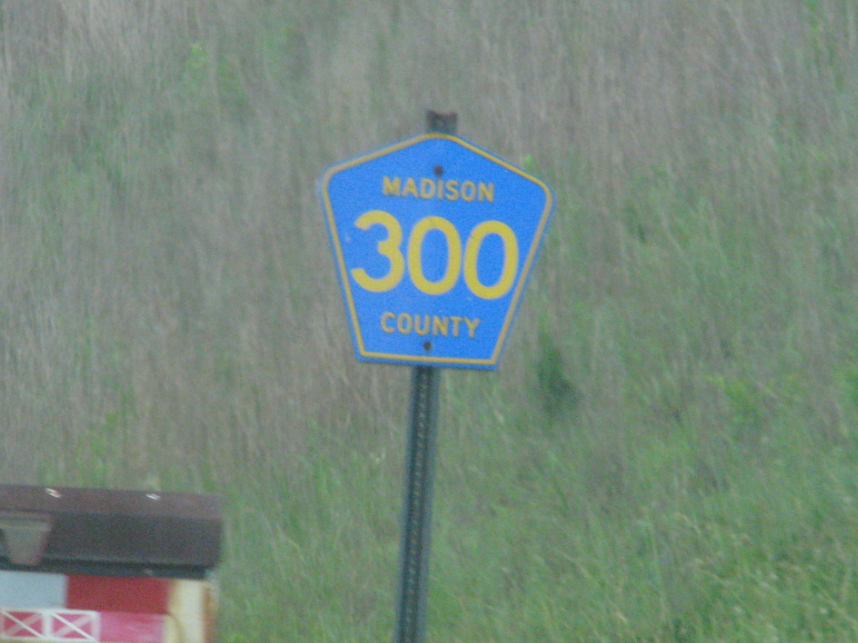This photograph captures a distinctive street sign indicating "Madison" with the numeral "300" beneath it, followed by the word "County". The sign is striking blue with yellow lettering and features a yellow border. Its shape is nearly diamond-like, with a flat bottom edge, and it is mounted on a green metal post with cutouts. To the bottom left of the image is a red and white structure topped with a brown roof. The background showcases a grassy field, transitioning from a tan hue in the upper left corner to a more vibrant green in the lower right corner, offering a serene rural landscape.